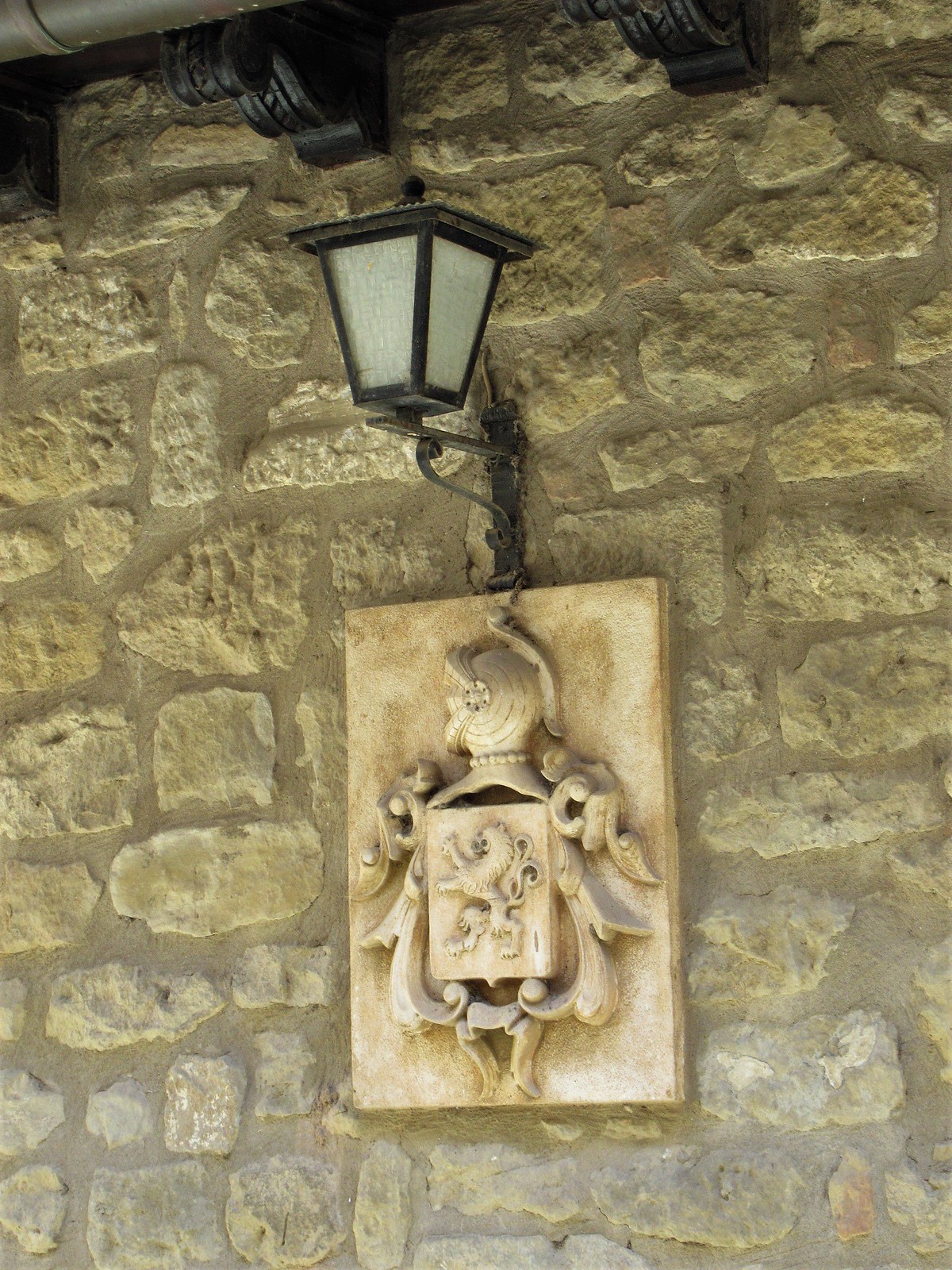This detailed image captures a stone carving embedded in a white-gray, possibly aged, stone wall. The carving, blending elements of tan and brown hues, features an emblematic design. At its center, a meticulously carved square showcases a lion motif. Surrounding this central square is a depiction of a Spartan or medieval knight's helmet with intricate designs, indicating a crest symbol often associated with door or entrance markings. The surrounding stone wall, characterized by both darker and lighter spots, enhances the antiquated feel of the scene. Above the emblem, there is a black lamp post, hinting at the vintage nature of both the lighting fixture and the stonework, suggestive of mid-20th-century craftsmanship. The entire composition presents a harmonious mix of stone and ceramic elements, underscored by the historical and decorative accents of the knight and lion.